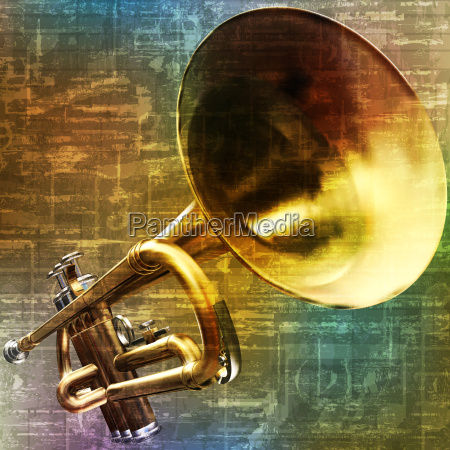This image features a highly detailed artistic rendering of a trumpet. The trumpet's bell, depicted prominently and quite large, emerges from the upper right corner and extends back to the center of the square image. The mouthpiece rests closer to the lower left corner, placing the instrument at a dynamic diagonal angle. The trumpet appears in a classic gold hue characteristic of brass instruments, with detailed touches such as a silver mouthpiece and three silver buttons for pressing.

The background is an abstract blend of various colors, including shades of golden-brown, copper, teal, purple, and light blue, which seem to transpose onto the trumpet itself, blending and adding complexity to its form. There's also a subtle incorporation of faded music notes, suggesting an overlay of music paper within the background's design. Text that reads "Panther Media," outlined in white, is centered in the image, though partially obscured by the intricate background patterns.

The trumpet’s artistic portrayal captures light and shading nuances, with the bell having brown tones at its top, effectively giving it a hollow, three-dimensional appearance. The handle of the trumpet shines with a reflective gold finish and features notable red and black bands. Overall, the image is a striking, visually complex composition that melds realistic trumpet details with an abstract, colorful backdrop.